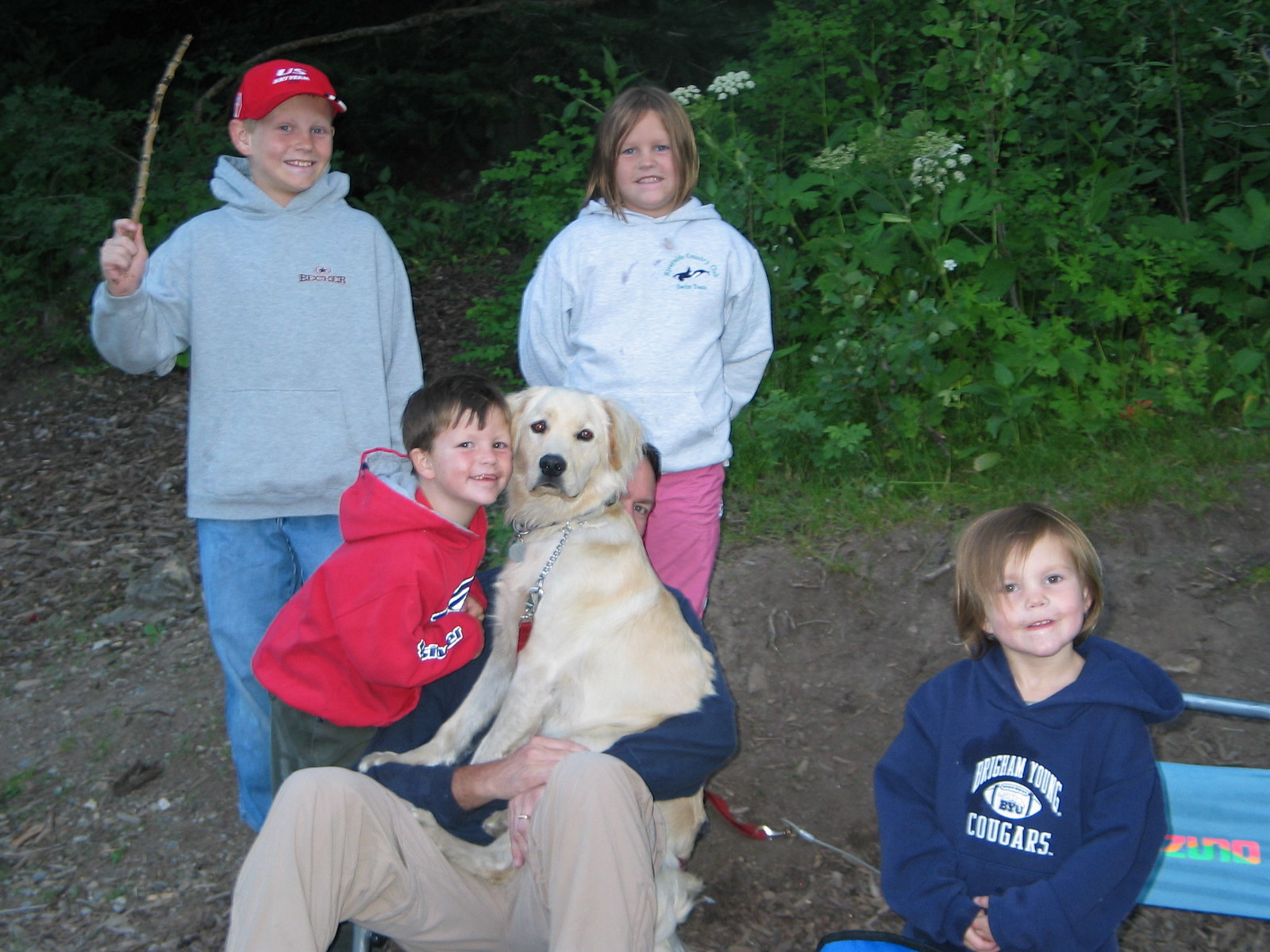The image captures a candid scene of a family camping trip set in a wooded area. At the center sits an older man in a low chair, partially obscured by a light-colored Labrador retriever sitting on his lap. The man, dressed in a blue sweatshirt and khakis, peeks out from behind the dog's neck, revealing a warm, gentle smile. To his left, a young boy, also smiling, nuzzles cheek-to-cheek with the dog. The boy is wearing a blue hoodie and green pants. Standing behind them are another boy and a girl. The boy, holding a stick like a bat, wears a red cap, a gray hoodie, and blue jeans. The girl beside him has on a gray hoodie with a blue logo and pink pants. Both have brown hair. On the right side of the image sits another young boy in a blue Brigham Young Cougars hoodie, with brown hair and hands clasped in front of him. He is seated in another small chair separate from the rest of the group. Around them is a backdrop of green shrubbery, weeds, and small plants under a canopy of trees, completing the idyllic outdoor setting.